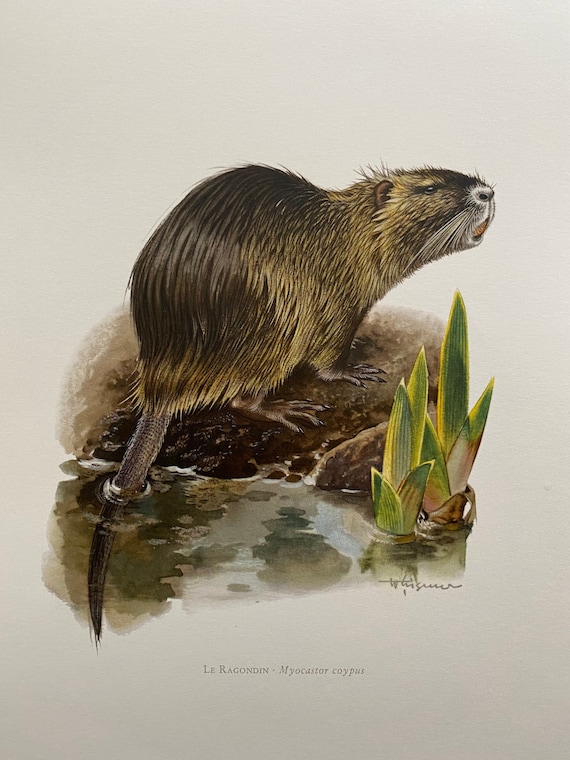The illustration is an antique print of a muskrat (sometimes referred to as a possum, beaver, or nutria) centrally positioned in a portrait orientation on grayish cream-colored paper. The muskrat, depicted in a lifelike manner with detailed features, has a wet, matted coat that transitions from deep brown on its back to a more golden tan color on its sides and head. Its face, characterized by small rounded ears, white fur around the mouth, and a black nose, is turned slightly upward and to the right, with its open mouth revealing a slightly yellowish hole, possibly its teeth. 

The muskrat is crouched on all fours atop a brown rock, which transitions from dark brown at the back to a lighter brown at the front, giving texture and depth to the scene. Its long, dark brown tail hangs down and partially submerges into the brownish water below. Adjacent to the muskrat on the right side of the composition, a group of vibrant green, pointed-leaf plants rise sharply from the water. Some of the plants show shades of light pink near their bases, adding a subtle contrast to the green foliage. Beneath the plant, a gray signature is visible, albeit too small to read clearly, and additional gray text stating "L-E-R-A-G-O-N-D-E-N hyphen M-Y-O-C-A-S-T-O-R-C-O-P-U-S" underscores the work. The background subtly transitions from light to dark gray, enhancing the antique aesthetic of the print.